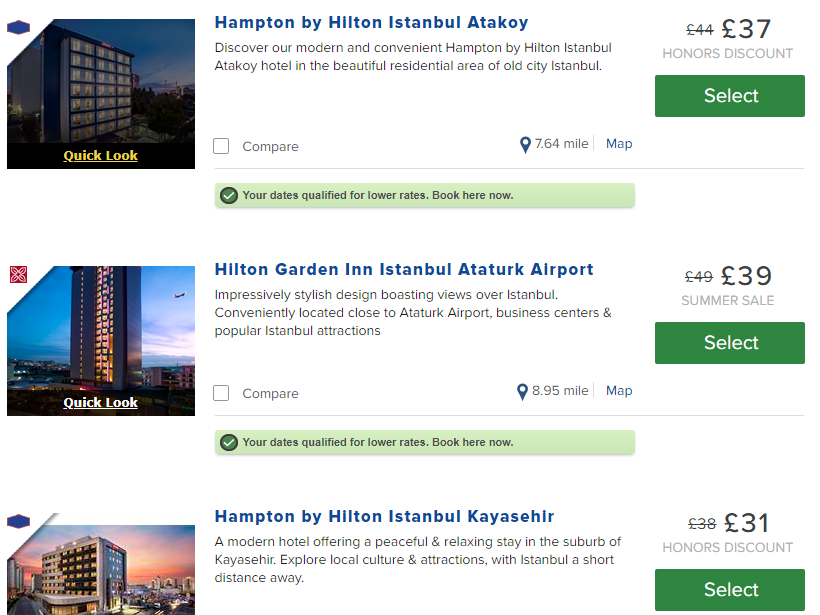**Detailed Caption:**

This is a detailed comparative image displaying search results for three hotels, showcasing their pricing and features. The image, approximately square in shape and set against a white background, lists the hotels vertically in a stacked format. 

Each hotel entry includes a thumbnail image on the left, with the hotel logo positioned in the upper left corner of the thumbnail. The hotel name is prominently displayed in blue font, followed by a detailed description in gray font. Additional links and buttons are provided for each listing, including options to compare, view distance from key locations, access a map, and view pricing details. 

1. **Hampton Inn by Hilton Istanbul Kadikoy**: 
   - **Description**: "Discover our modern and convenient Hampton by Hilton Istanbul Kadikoy Hotel in the beautiful residential area of Old City Istanbul."
   - **Details**: The hotel exudes a straightforward charm, ideal for travelers seeking modern amenities in a historic setting.
   - **Price**: 37 (currency unit).
   - **Features**: Includes a "Select" button in a green rectangular box.

2. **Hilton Garden Inn Istanbul Atatürk Airport**:
   - **Description**: "Impressively stylish design boasting views over Istanbul, conveniently located near Atatürk Airport, business centers, and popular Istanbul attractions."
   - **Details**: This hotel combines stylish design with convenience, perfect for business and leisure travelers.
   - **Price**: 39 (currency unit).
   - **Features**: Positioned with a green "Select" button at the bottom.

3. **Hampton by Hilton Istanbul Kayaşehir**:
   - **Description**: "A modern hotel offering a peaceful and relaxing stay in the suburb of Kayaşehir, with local culture and attractions in Istanbul a short distance away."
   - **Details**: This hotel provides a serene environment, ideal for those wishing to explore local culture from a tranquil base.
   - **Price**: 31 (currency unit). 
   - **Features**: Comes with a green "Select" button for booking.

Each hotel listing is separated by buttons and links that facilitate easy comparison and map viewing. The clear organization and detailed descriptions provide travelers with a comprehensive view of their options, assisting them in making an informed decision.